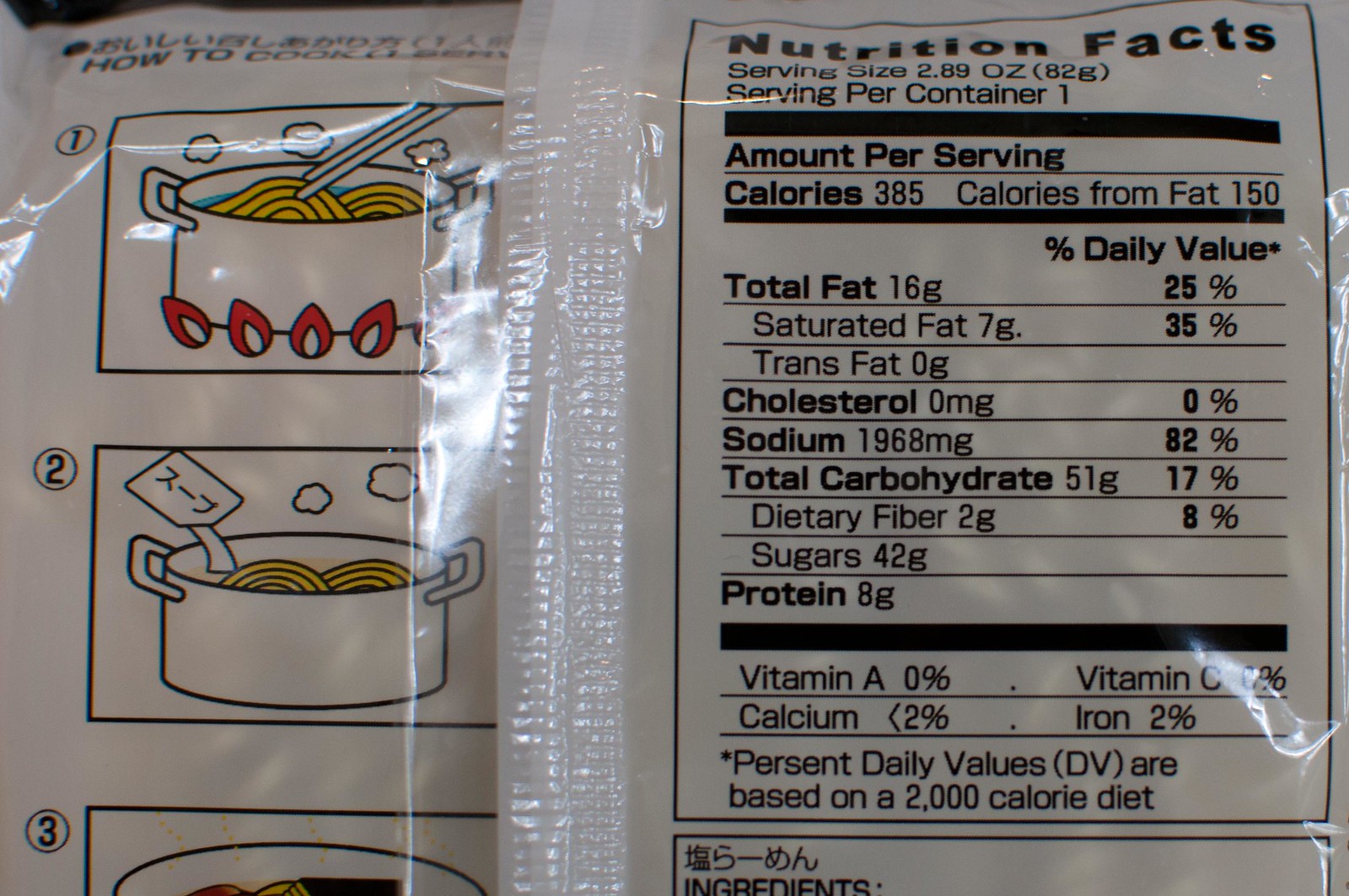This photograph depicts the back of a plastic packet of instant noodles. On the left side, there are illustrated cooking instructions. At the top, a label reads "how to," followed by step-by-step visuals. Step one, marked with a number 1 in a circle, shows a pot with noodles and water over a flame, emitting steam. Step two, similarly marked with a number 2, illustrates seasoning being poured into the pot. There's a partial view of step three, which is not fully visible. The right side of the packet displays the Nutrition Facts label: serving size is 2.89 ounces (82 grams), with one serving per container. The label states that each serving contains 385 calories, including 150 calories from fat. Nutritional details follow: Total Fat is 16 grams (25% DV), with Saturated Fat at 7 grams (35% DV) and no Trans Fat or Cholesterol. Sodium content is high at 1968 milligrams (82% DV). Total Carbohydrate is 51 grams (17% DV), including 2 grams of Dietary Fiber (8% DV) and 42 grams of Sugars. Protein content stands at 8 grams. The vitamin and mineral content includes 0% for both Vitamin A and C, less than 2% Calcium, and 2% Iron. An asterisk notes that Percent Daily Values (DV) are based on a 2000 calorie diet.